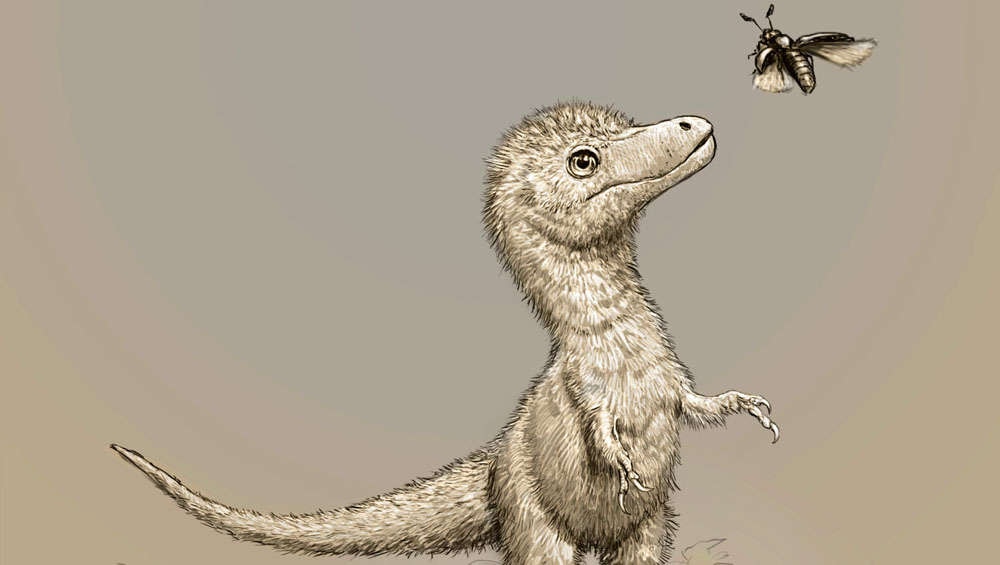In this detailed and slightly animated black and white drawing against a beige background, a small, fluffy theropod dinosaur stands on two legs, covered with short, downy feathers that hint at its youth. The dinosaur's overall form is reminiscent of a tiny T-Rex, complete with a long tail extending behind it and tiny, fuzzy arms ending in three claws each. With its large, expressive eye, the dinosaur gazes up curiously at a sizeable insect, likely a moth, hovering nearby. The insect, notable for its dark body with white specks and filmy wings, is about half the width of the dinosaur's head and just within reach, capturing the creature's full attention as it appears ready to chase or interact with its airborne companion.